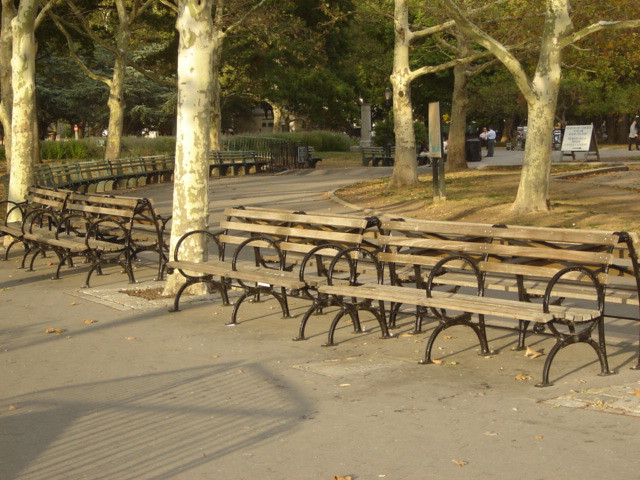In this vibrant park scene, multiple light tan brown wooden benches with ornate black iron legs and armrests are neatly lined up along a looping gray stone path. This path winds from the right to the left and back around to the right within the park. The benches are interspersed with majestic white and brown trees with green leaves at the top, casting gentle shadows on the ground. Scattered autumn leaves in hues of brown, orange, and red add a seasonal touch, contrasting with the patchy green grass and brown dirt behind the benches. In the background, a white sign with lettering can be seen, hinting at an event, and a man in a white shirt and dress slacks converses with a woman, adding life to the serene setting. The sun shines brightly, enhancing the overall warmth and inviting atmosphere of the park.